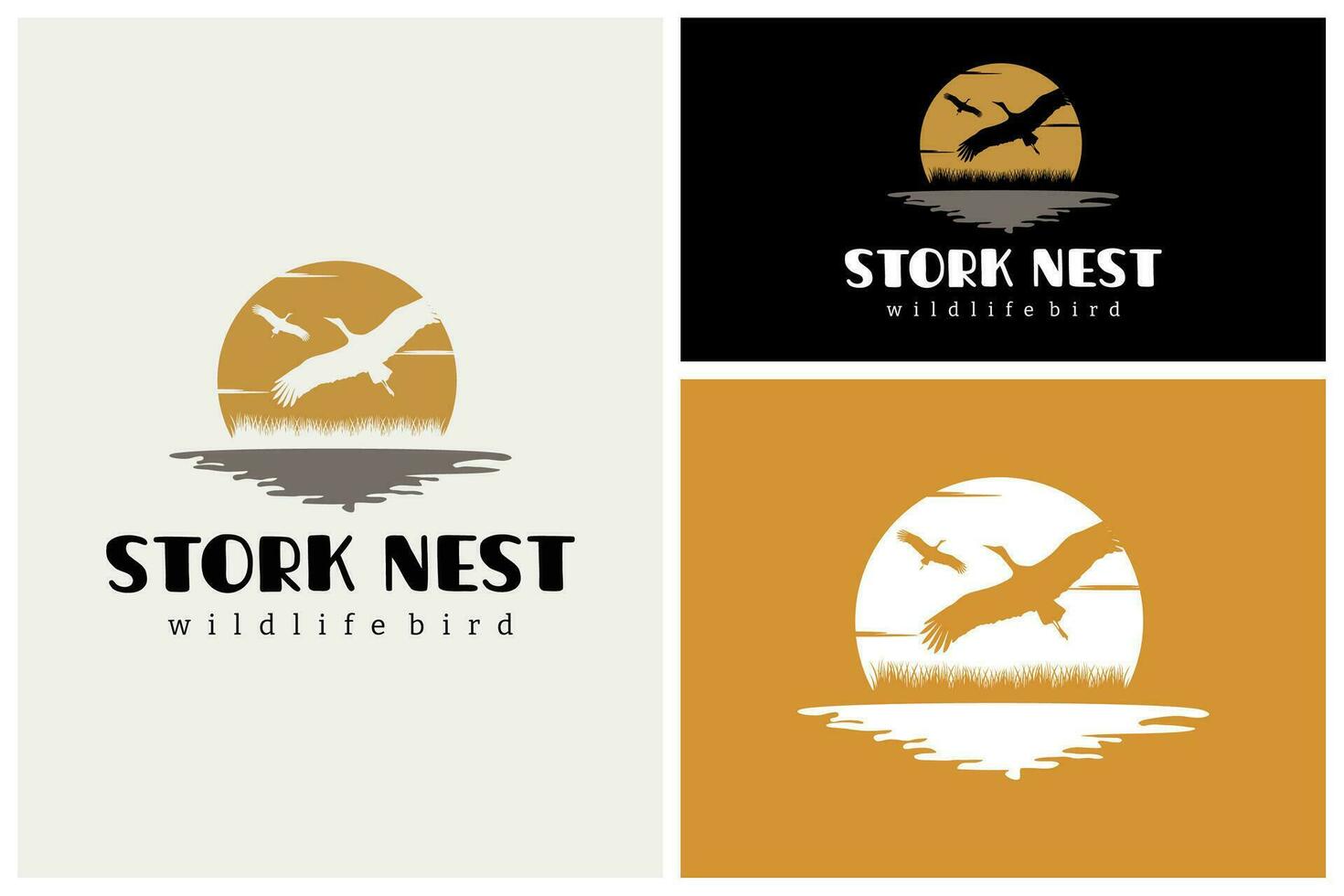The image showcases a series of three logos on different backgrounds, illustrating variations of the "Stork Nest, Wildlife Bird" design. On the left side, the largest panel features a cream-colored background with the logo in black print depicting the words "Stork Nest, Wildlife Bird." The logo itself consists of an orange sun setting over a gray splash of water at the bottom, framed by tall grasses and two white birds flying, all in an upside-down triangular shape.

To the right, the upper panel is set against a dark black background, retaining the same logo but with variations in color: the sun and birds are orange, the grasses and splash of water remain gray, and the text "Stork Nest, Wildlife Bird" is now in white print. 

The bottom-right panel features an orange background with the same graphical elements but with no text. Here, the sun is depicted in white, while the birds and grasses are in orange, and the water splash is also in white. This multi-panel layout appears to be a promotional material, highlighting the versatility of the logo across different color schemes.